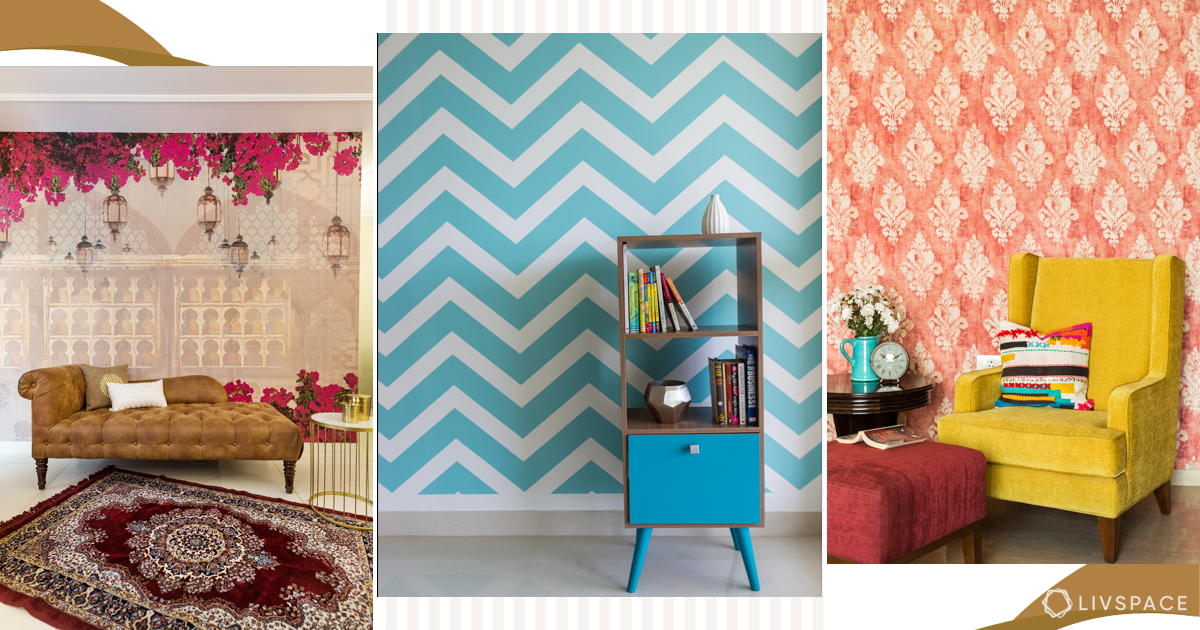The image depicts a stylish interior design layout, divided into three sections, each showcasing unique home decor arrangements. 

On the far left, a cozy scene features a brown velvet futon adorned with two pillows, paired with a deep red and white Persian-style rug. The backdrop includes an ornate wallpaper that gives the illusion of a building with bright pink bougainvillea flowers and hanging lanterns, complemented by a small gold and white table.

The central section displays a striking blue and white chevron-patterned wall. In front stands a small, elegant cabinet with a bottom drawer and four blue legs. The cabinet's shelves are occupied by books and knickknacks, topped with a silver vase, all set against a pristine white floor. Adjacent to this, there's a brown chaise lounge couch against a plain white wall with pinkish floral accents.

The rightmost section highlights a mustard yellow velvet armchair with a multicolored cushion. In front, an ornate reddish-brown footstool holds an open magazine and is captioned “L-I-V-E-S” in brown text beneath it. This corner is complemented by red and white fleur-de-lis patterned wallpaper. Adjacent to the chair is a small brown wooden table with white flowers in a blue pot, alongside a clock.

Each section embodies distinct decorative elements, yet together they convey a cohesive, vibrant aesthetic suitable for a home decor magazine or online shopping platform. The bottom watermark reads "Live Space," unifying the sections into a single, curated presentation.